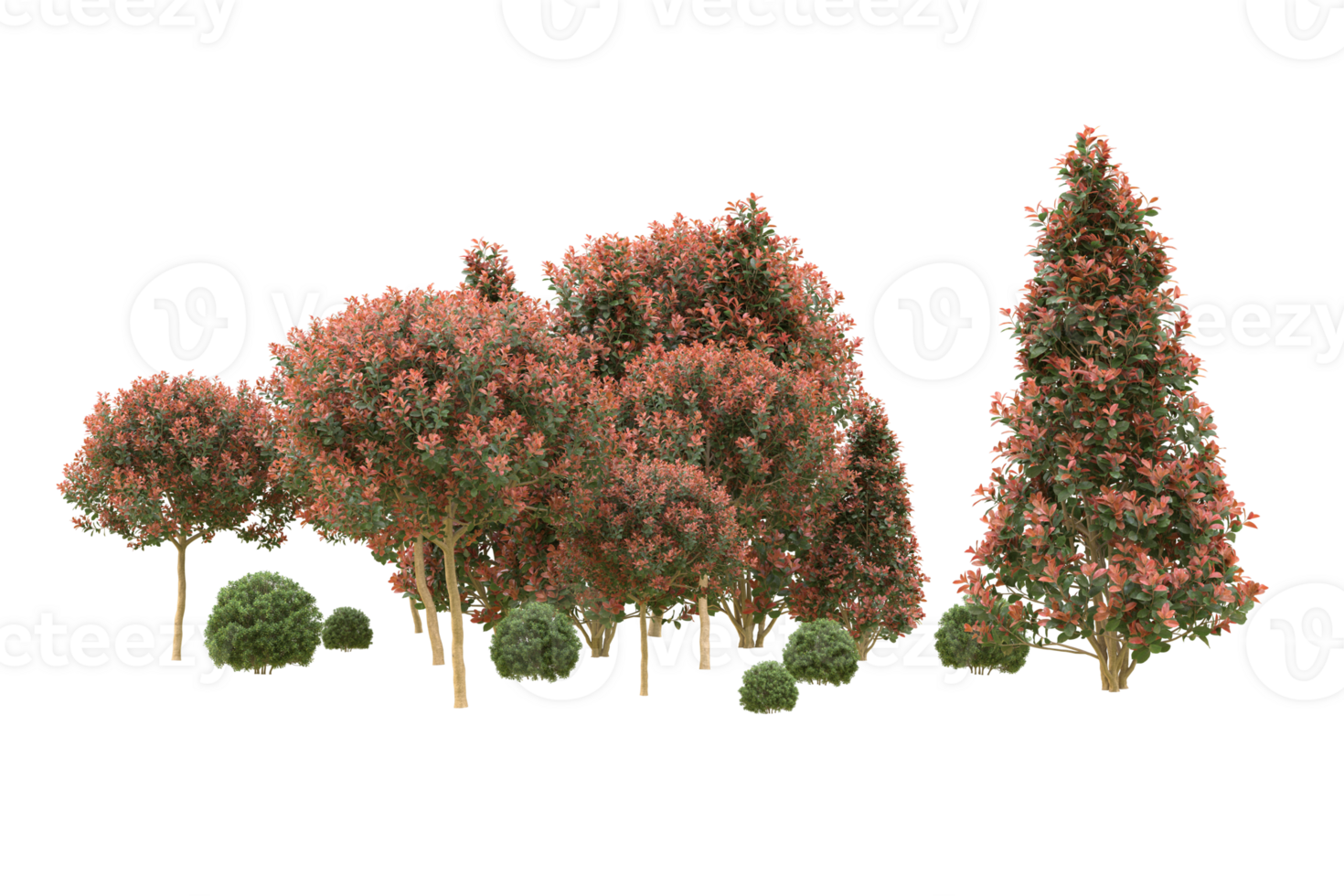In this image, there are about a dozen well-manicured trees set against a solid white background. The trees have a light brown to yellowish-brown trunk and exhibit two distinct shapes: rounded and Christmas tree-like. The foliage is a mix of vibrant green and light pinkish-red to salmon-colored leaves and flower petals. These colors create a striking visual contrast. The trees with the rounded shape have a more circular arrangement of fine green and pinkish leaves, while the conical, Christmas tree-shaped ones feature similarly colored leaves arranged in a triangular pattern. Additionally, there are small green shrubs at the base of the image, which appear to be young trees. A watermark with a "U"-shaped logo and the text "Vecteezy" is present in the background, indicating the source of the image.